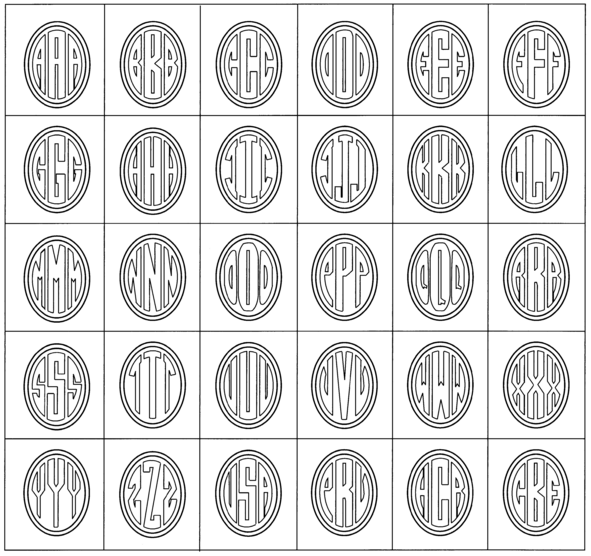This black and white photograph features a grid layout, structured with five rows and six columns, forming a total of 30 squares. Each square contains a circular monogram pattern, where the central letter is the largest and flanked by two smaller, identical letters, all in a block font. This repeating design starts with "AAA" in the first square, followed by "BBB," "CCC," and continues sequentially through the alphabet until "ZZZ." Notably, beyond the alphabet, the bottom row includes unique combinations such as "USA" and "CBE," suggesting these might be intended for cutouts or labeling purposes.